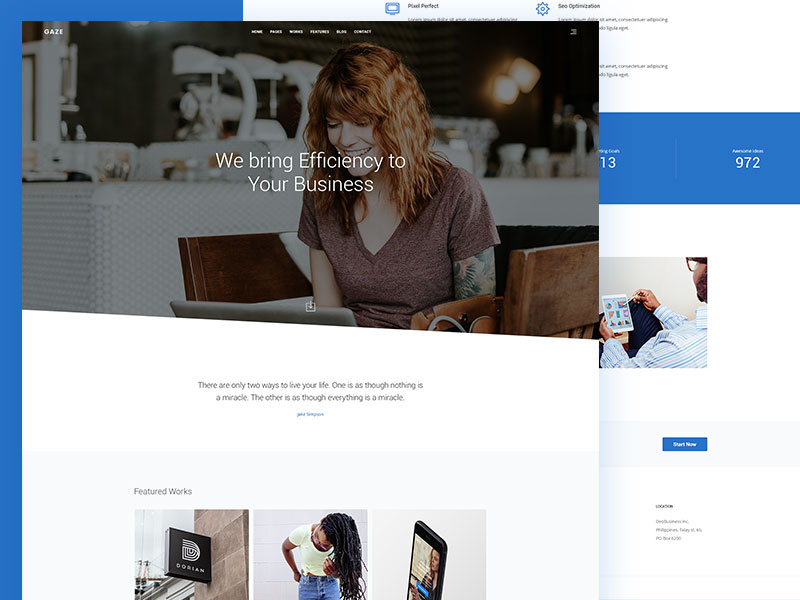This collage showcases multiple screenshots from the same website, intricately layered to highlight different design elements. In the background, on the left side, there's a webpage characterized by a blue border along its left edge and top. Overlapping this, on the right side, is a second webpage screenshot, positioned in such a way that it partially covers the first one. Further overlaying this second screenshot, towards its left side, is a third screenshot. This final, fully visible screenshot prominently features a woman typing on a computer as its background image. Superimposed on this background is the text "We bring efficiency to your business." Below this text, a brief paragraph in gray font provides additional information. Near the bottom of the screenshot, the text "Featured Works" appears at the top left corner, accompanied by small thumbnail images beneath it. These thumbnails depict a business sign, a woman walking down the street, and a cell phone, respectively.